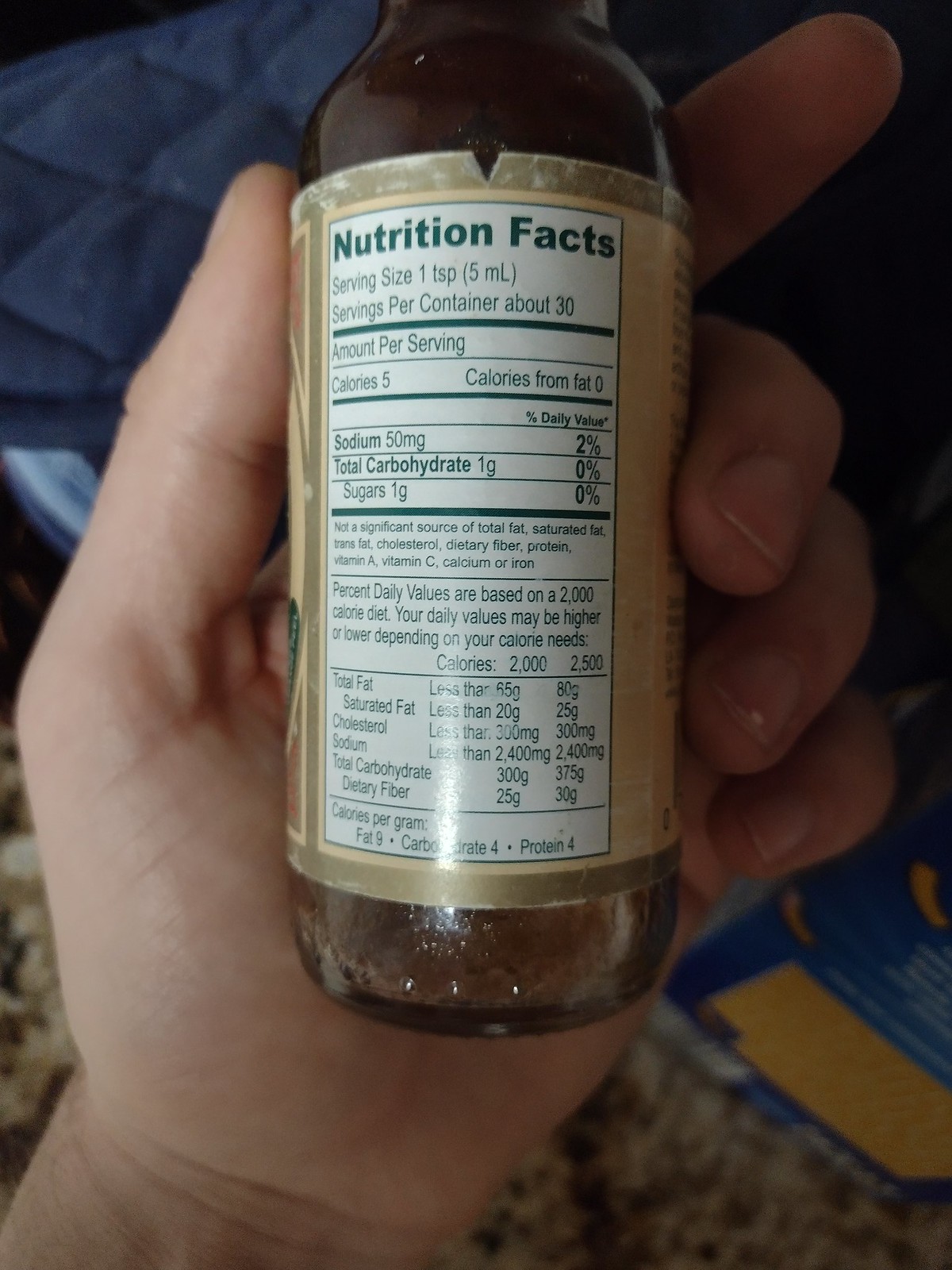In this detailed photograph, a person is holding a glass bottle containing a brownish liquid with their left hand. The bottle's label features a mix of golden, yellow, tan, brown, white, and black colors. Prominently displayed on the label is a Nutrition Facts panel with green text on a white background, detailing that each serving size is one teaspoon (5 ml), with about 30 servings per container. Each serving provides 5 calories, 50 milligrams of sodium, 1 gram of carbohydrate, and 1 gram of sugar. Unfortunately, the image does not clearly reveal the specific ingredients. Additionally, below the hand holding the bottle, a blue cloth object is visible, as well as what appears to be an orange and blue box. The scene also includes a partial glimpse of a tan, black, and white-colored countertop.